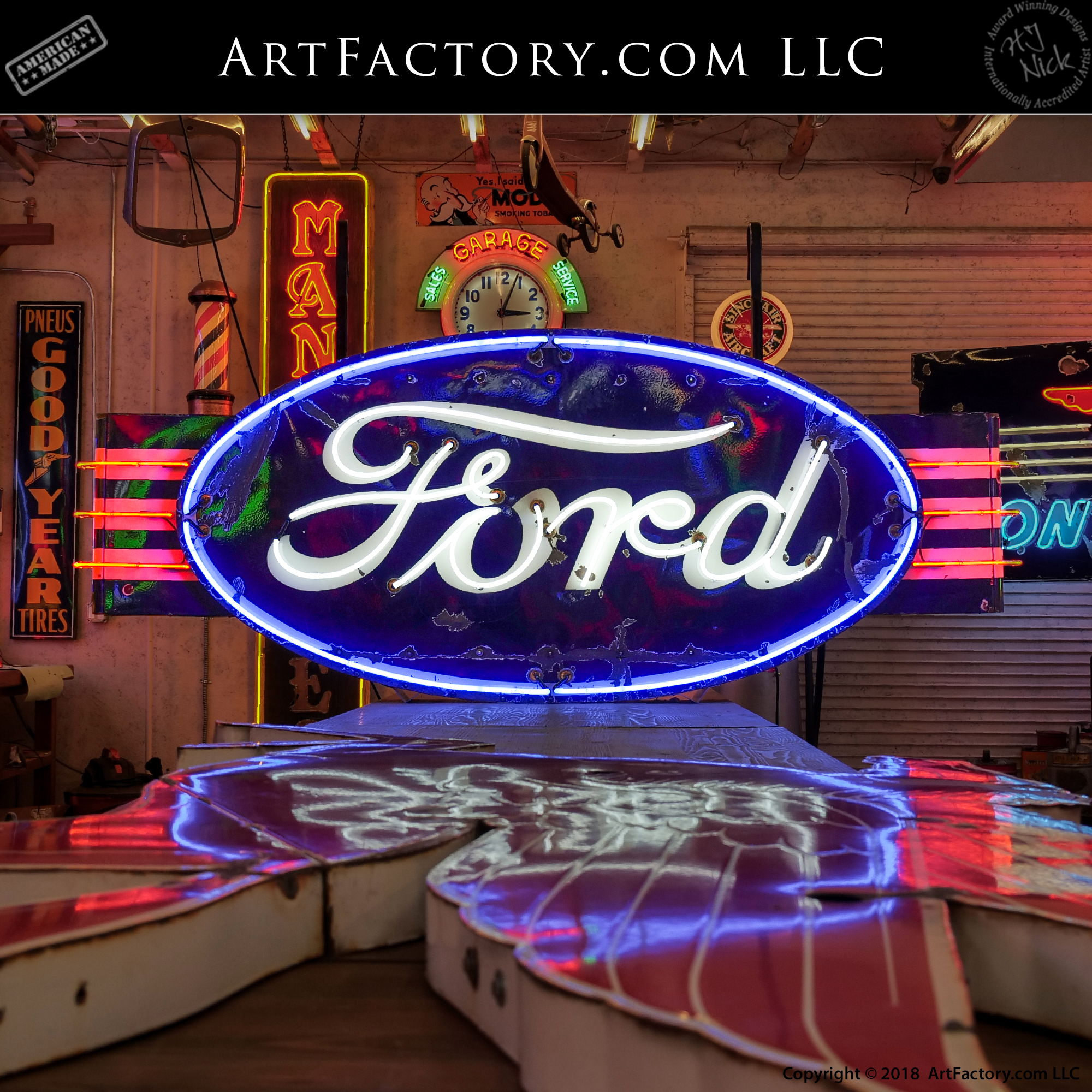The photograph, presented as an advertisement for ArtFactory.com LLC, captures an elaborate indoor scene brimming with nostalgic Americana and neon craftsmanship. Dominating the center is a large, elliptical blue neon sign emblazoned with the iconic Ford logo in white script, enhanced by a surrounding neon border. This central piece mirrors on a reflective tabletop surface below. 

The backdrop, a cement wall, is adorned with a variety of neon signs, including a prominent Goodyear Tires sign and another partially obscured sign starting with "M-A-N." Also present is a nostalgic barbershop spiral and a clock labeled "Garage Services," framed with green and orange neon lights. Additional elements like the grill of a vintage 1920s car and a suspended scooter add to the automotive-themed decor. 

A non-illuminated but large neon sign rests on the ground, showcasing red, wing-like designs with white sides. The upper part of the image includes a black header with the company's branding: "ArtFactory.com LLC" prominently in white, accompanied by "American-Made" within an angled white box on the left, and a circular insignia on the right proclaiming "Internationally Accredited Award-Winning Designs" around "H.J. Nick." The bottom right corner notes the copyright year, "2018 ArtFactory.com LLC" in black text.